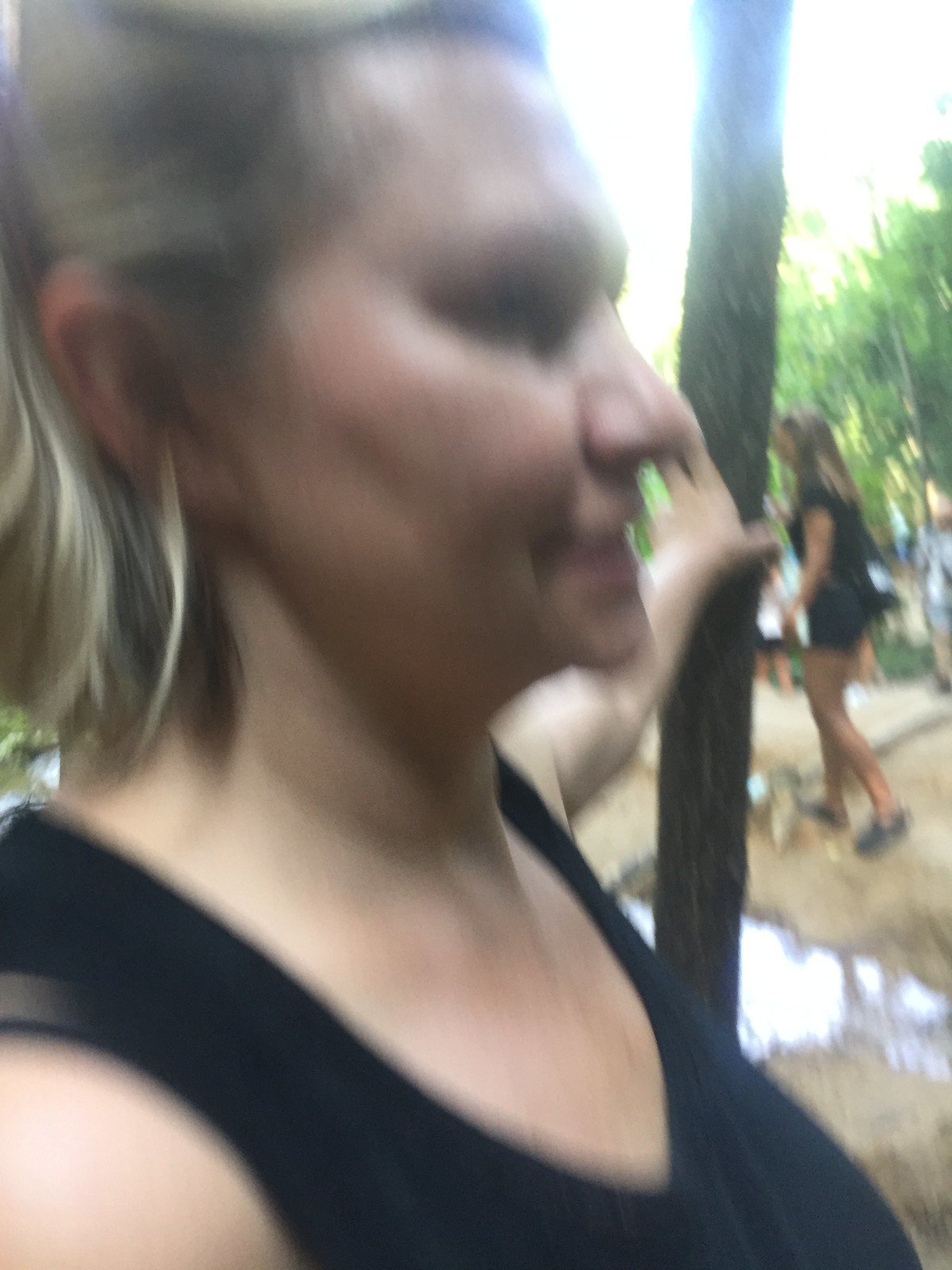A very blurry photograph captures a woman from her profile, facing to the right. Her face and the area just below her neckline are visible. Her left arm is outstretched, grasping what appears to be a tree or wooden post in the background. She has short, shoulder-length dirty blonde hair and is dressed in a black tank top. The woman appears to be in her 40s. In the background, another woman is seen walking to the left with her side and back facing the camera. She is wearing dark-colored shorts and a tight dark-colored t-shirt. Behind her, trees are illuminated by sunlight from above, and the ground underneath features dirt and possibly a puddle reflecting the light.